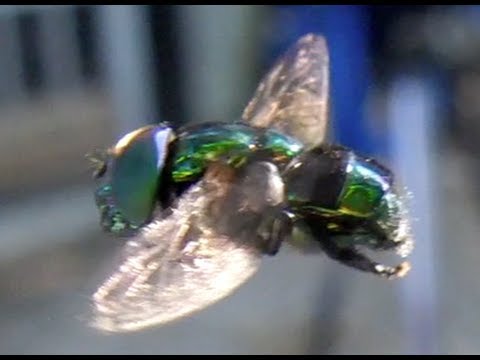In this close-up photograph, a fly is captured in mid-air, its body displaying vibrant emerald green hues from head to rear. The wings, outstretched in flight, appear silver and are as wide as the fly's body. The photograph, while slightly blurry, suggests the fly is in motion, making it difficult to discern intricate details in the wings and segmentation. The fly's head exhibits a smooth, metallic shine, possibly greenish-gray depending on the angle of light. The background is entirely blurred, providing no discernible features, which enhances the focus on the fly's iridescent and colorful appearance. The overall image is reminiscent of a painting against a dark to light blue gradient backdrop.